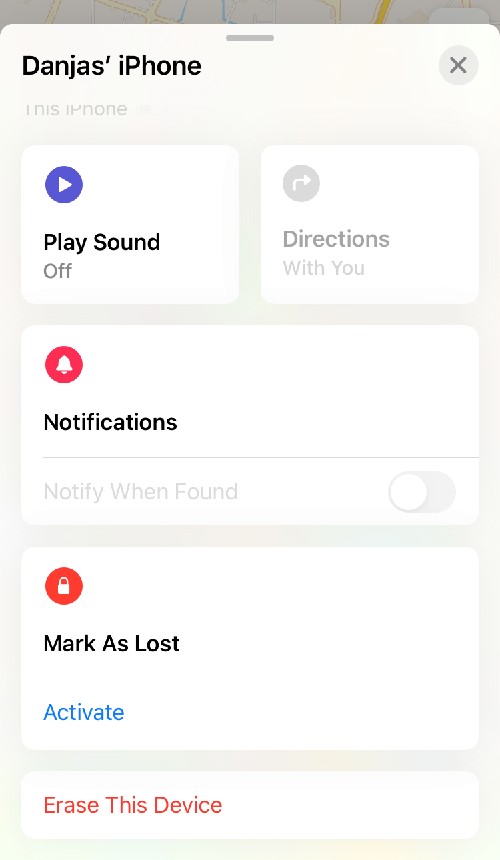A screenshot taken on an iPhone displaying the "Find My iPhone" interface. The header prominently features "Danja's iPhone" in bold black letters at the top left corner, with a gray "X" on the upper right for closing the window. The overall background is a very light gray tone. Below the header, the text "This iPhone" is displayed.

Several interactive boxes are present on the screen. The top-left box labeled "Play Sound" is highlighted with a purple circle containing an arrow, indicating a clickable play button, though the sound function is currently off. Adjacent to it, the "Directions with You" box appears grayed out and is not active.

Below these, a full-width box labeled "Notifications" features a red circle with a white bell icon to the left. The text "Notify When Found" appears alongside it, but this option is turned off and grayed out.

Further down, a red circle with a white lock icon represents the "Mark As Lost" feature, with bold black letters stating the same. The option to activate this feature is shown in red text as "Activate."

In a distinct, narrow section at the bottom, the "Erase This Device" option is displayed in red, indicating the user's ability to remove all data from the iPhone if necessary.